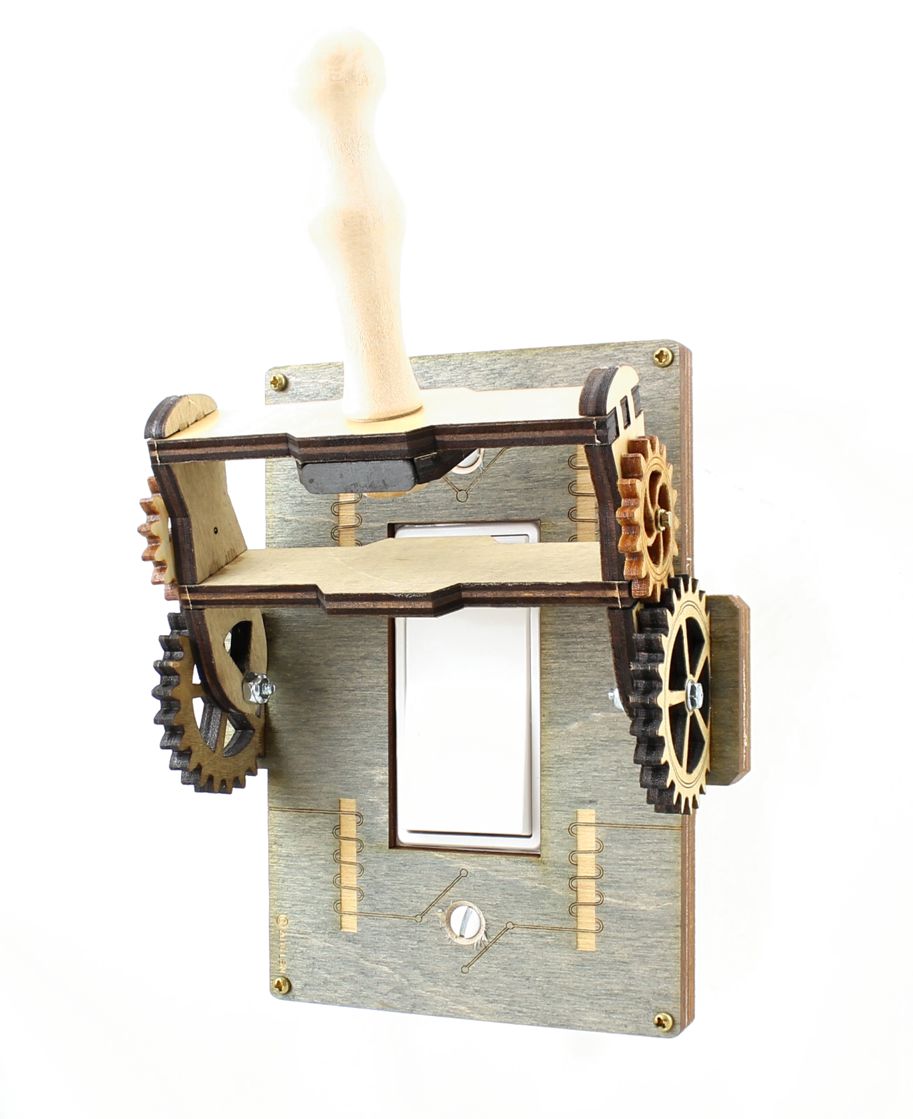The image depicts a highly detailed and creative light switch cover, designed to resemble a mechanical device. The light switch itself is a broad, rocker-style switch, colored in white. This switch is fitted with an intricately laser-cut wooden panel that overlays the existing switch plate. The panel is accentuated with an array of gears and other mechanical elements. Specifically, there are two large gears on either side, each accompanied by smaller gears above them, contributing to a complex design akin to a Rube Goldberg machine.

The panel includes a sculpted handle at the top, crafted from wood in various tones, ranging from light tan to a darker brown, possibly made from balsa wood or thin luan plywood. When the handle is pulled down, it interacts with the gears, which align to push the light switch on or off. This motion is supported by two horizontal wood pieces that frame the handle. The laser-cutting process has also imparted decorative designs burned onto the wood, adding to its aesthetic appeal.

The panel is mounted onto the wall over the existing light switch plate with four brass screws, one in each corner, providing stability and a polished finish. In the center of the panel, rectangular notches are surrounded by decorative lines, contributing to its ornate appearance. The background of the wooden cover is a light gray, contrasting with the various wood tones and making the entire structure a fascinating and functional piece of art.